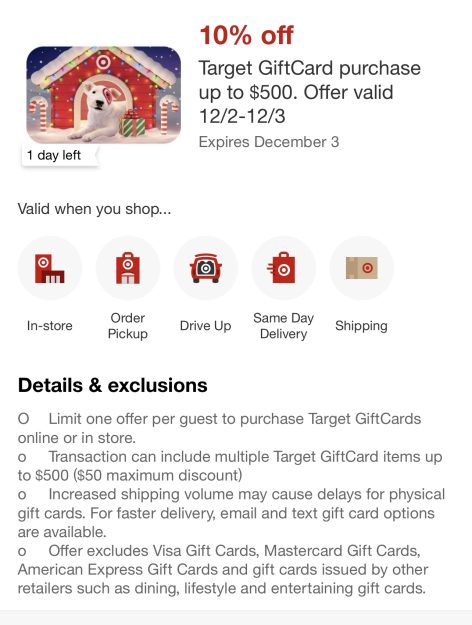Screenshot of a promotional offer from Target: The image features a 10% off discount displayed in bold red text at the top. This discount applies to Target gift card purchases up to a maximum of $500, and is valid from December 2nd to December 3rd, expiring on December 3rd. The visual includes a festive scene with a doghouse adorned with Christmas lights and flanked by two candy canes, housing the iconic Target dog with the Target emblem atop the house. The offer highlights several purchasing options including in-store orders, pickup, drive-up, same-day delivery, and shipping, each accompanied by the Target logo. The promotion details mention that there are specific exclusions and a limit of one transaction per gas purchase, with a maximum inclusion of $500 per transaction.